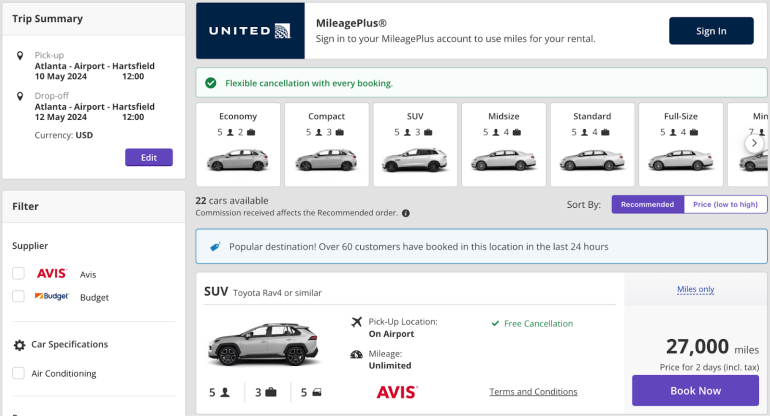This is a screenshot of a website likely belonging to an auto rental service, prominently branded with the name "United" at the top and featuring "MileagePlus." The site instructs users to sign in to their MileagePlus account to use miles for their rental. A noticeable "Sign In" button is present for user access. 

On the left side of the screen, there's a trip summary indicating a pick-up at Atlanta Airport Hartsfield on May 10, 2024, at 12:00 PM, and a drop-off at the same location on May 12, 2024, at 12:00 PM. The pricing currency is listed as US Dollars, with buttons available for editing trip details and filtering rental options by supplier, car specifications, and air conditioning.

Centrally located at the top of the page are category options for vehicle types, including Economy, Compact, SUV, Midsize, Standard, Full-size, and Minivan, with a note about flexible cancellation policies for every booking.

At the bottom of the screenshot, there is a highlighted option for an SUV with 27,000 miles on it, accompanied by a "Book Now" button, encouraging immediate reservation.